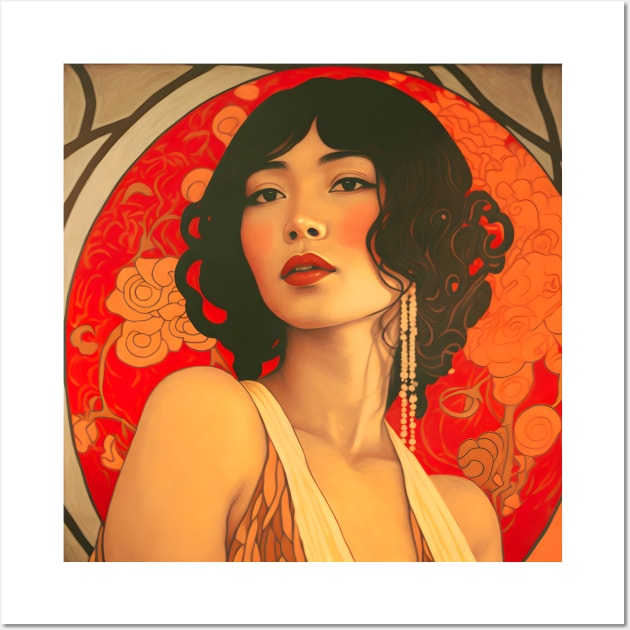This realistic painting or illustration showcases an Asian woman facing forward with her head slightly tilted to the left over her shoulder. She has short, curly black hair that falls above her shoulders, and her almond-shaped eyes taper widely at the ends. Her facial features include a very small, pointy nose, red lipstick, and rouged cheeks. She has light yellowish skin and is adorned with one long, dangling bead earring, resembling seed pearls, that extends from under her hair down to her shoulder. She is dressed in a sleeveless, strapped dress with a deep V-neck that features a white base adorned with yellow and gold designs transitioning to peach, red, and light orange hues. Behind her is a red circular screen with elaborate white, red, pink, tan, and peach-colored floral patterns, adding depth and richness to the scene. The image captures her from the head down to the chest, where her arms are cut off in the picture.